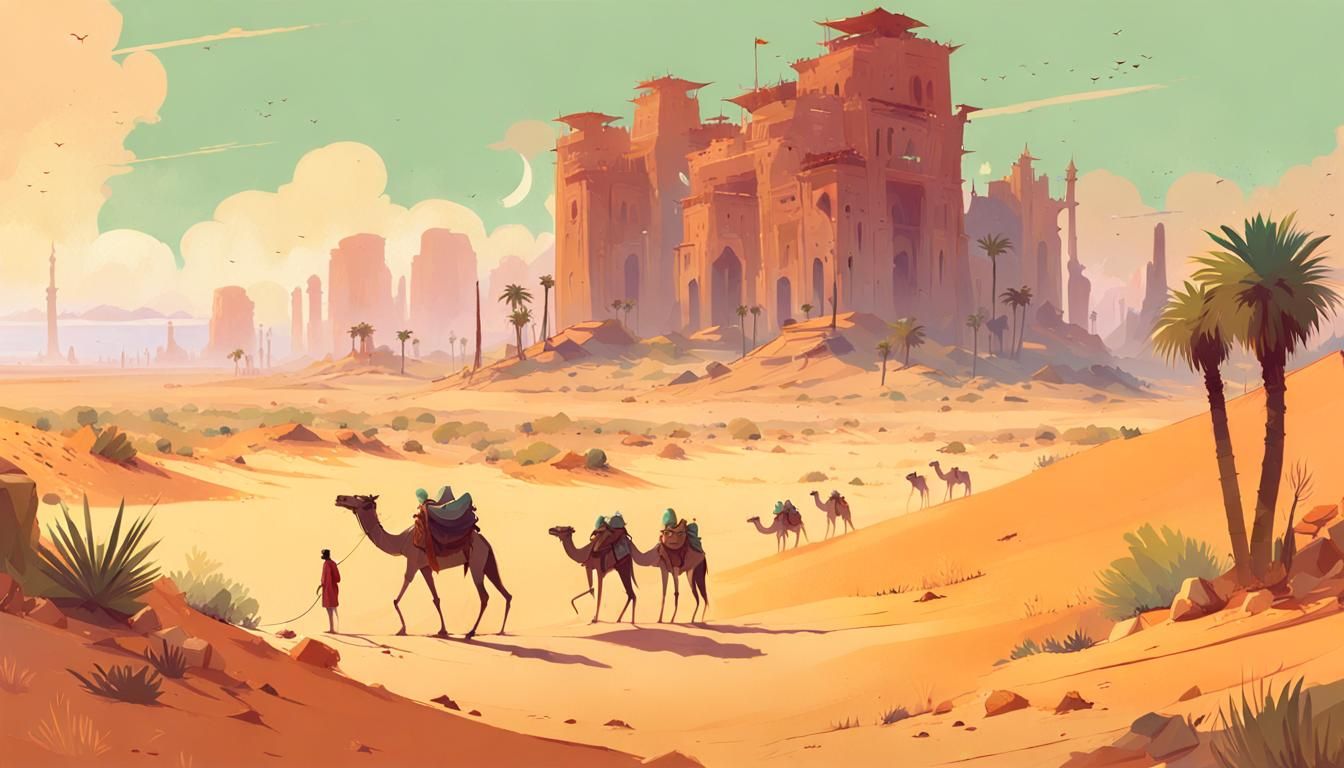The image is a detailed illustration of a lively desert scene. At the forefront, a man dressed in a red tunic is leading a camel; nearby, to his right, two other camels are laden with packs. Several more camels stretch into the distance. Dominating the right side of the scene is a large, clay-colored building that resembles a palace, with surrounding mounds of sand and a cluster of green and yellow palm trees. Further to the left, the scene fades into the hazy distance where more buildings can be glimpsed. In the bottom left corner, a hill dotted with scrubby desert plants can be seen, which rises again on the right side where a palm tree stands. The sky above is painted a light teal blue with streaks of big white clouds casting a yellowish tone over the landscape. The vast expanse of tan sand dunes is interspersed with occasional cacti and rocky formations in various hues of brown, pink, white, and yellow, adding texture to the arid tableau.